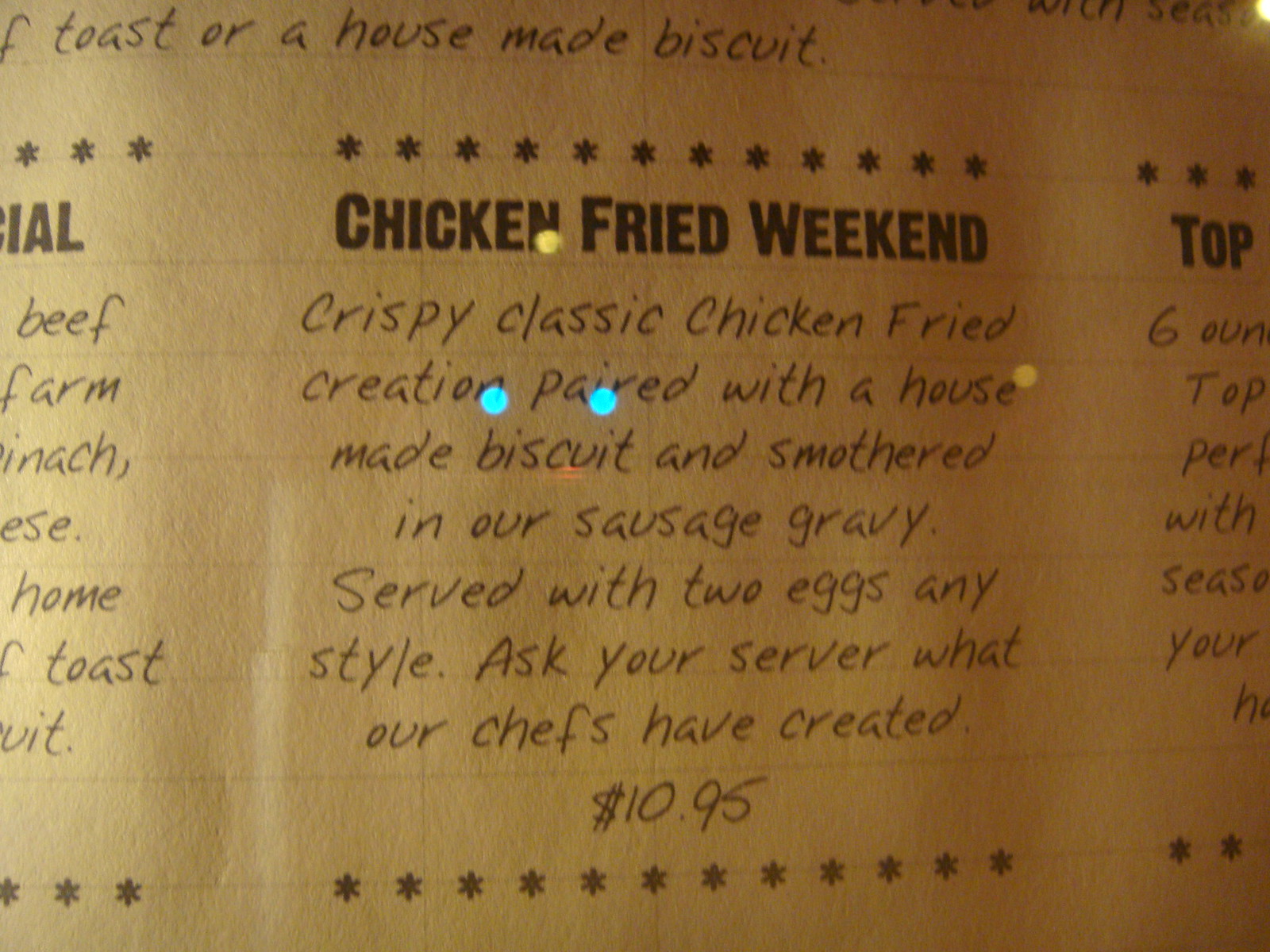This photograph captures a small portion of a restaurant menu displayed in a typeface that mimics handwriting. The section highlighted presents an offering labeled "Chicken Fried Weekend." Above this title, the menu indicates that choices include toast or a house-made biscuit, separated by a line of vintage typewriter-style asterisks.

The description reads: "Crispy classic chicken fried creation paired with a house-made biscuit and smothered in our sausage gravy. Served with two eggs, any style. Ask your server what our chefs have created. $10.95." Intriguingly, amidst this handwritten-style typeface are small, colored circles of light: a yellow circle embedded within the word "and," and two blue-green circles around "creation" and "paired." Another yellow circle of light is seen off to the side. These spots, about the size of an 'E' in the text, add a unique visual element to the menu.